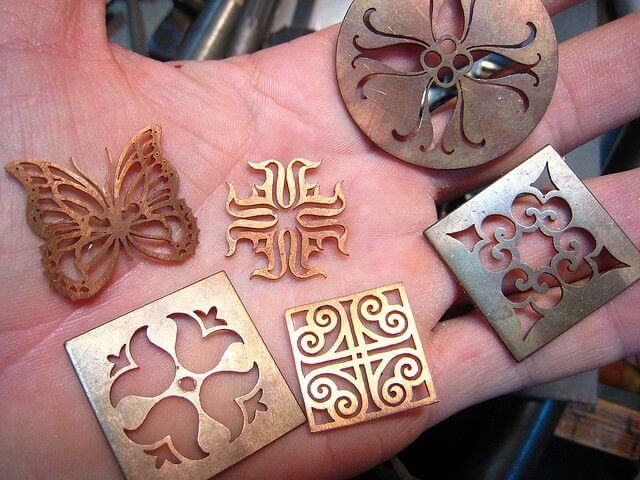In the image, a left hand, palm open, belonging to what appears to be a white male, delicately cradles six intricately designed metallic emblems. The emblems, varying in size and shape, showcase detailed craftsmanship in materials resembling copper and brass. 

Starting from the left, there's a bronze-colored butterfly, complete with detailed antennas and vein-like impressions on its wings. Adjacent to it, positioned just below, is a square emblem with flower petals intricately engraved, resembling a four-leaf clover, cut out from copper. In the center, there’s an ornate object featuring a symmetrical design of duckbill-like shapes facing in four directions, reminiscent of flames or crests. Moving downwards, another square emblem appears, this one characterized by curlicue patterns creating an impression similar to an eight-pointed star with arrowhead details at the corners. To the right of this, closer to the index finger, a square emblem showcases a unique motif of scroll patterns, leading to a small central square, all reflected in polished brass. Finally, at the top right, a circular emblem displays an elegant arrangement of tulip-like shapes with a central diamond figure, carved in a darker brass or copper material.

The emblems rest just below the fingers, providing contrast against the skin, and their delicate, detailed engravings highlight the craftsmanship involved in their creation.